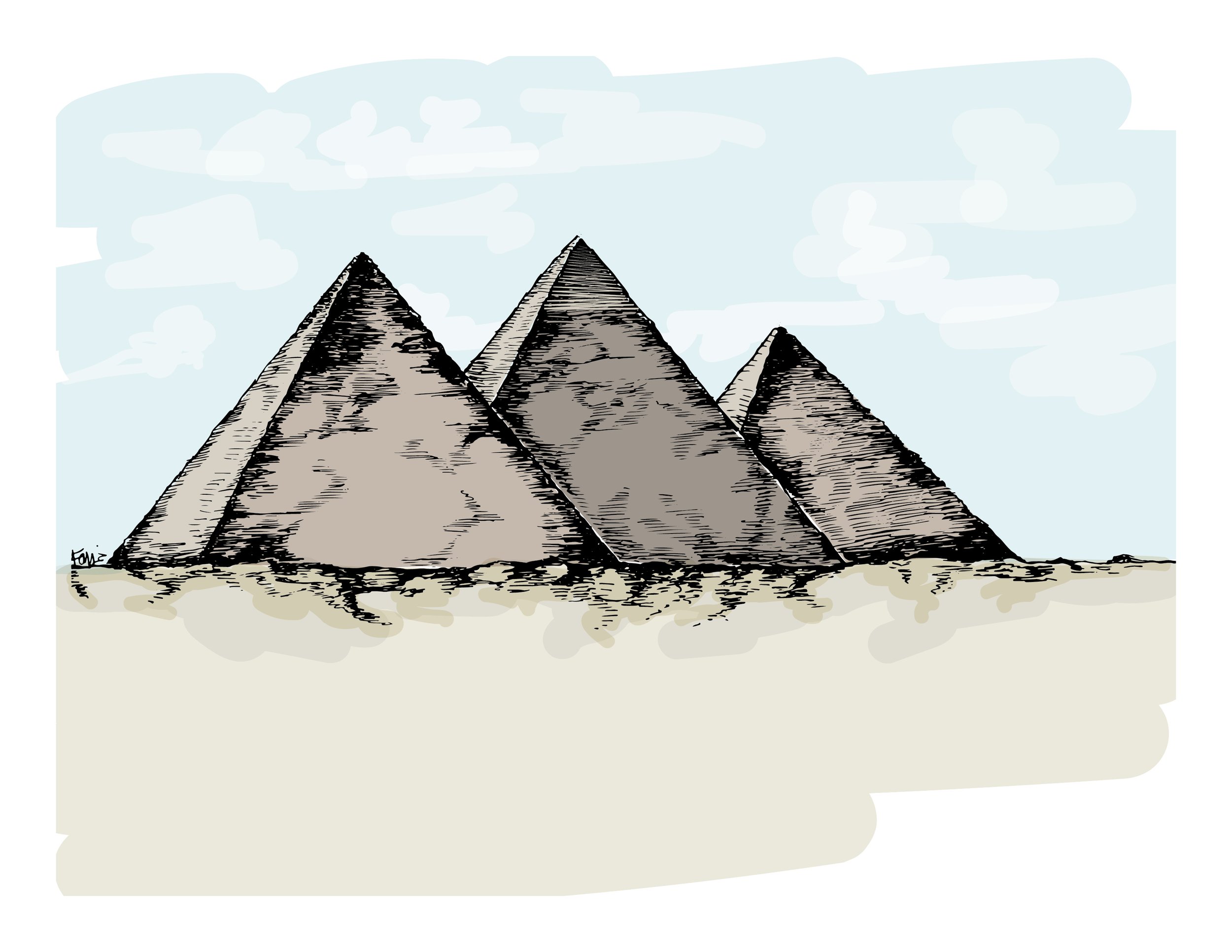This image is a detailed artwork featuring three pyramids, rendered using a combination of ink and watercolor techniques. The left pyramid, positioned in the foreground, stands in front of the other two pyramids. The middle pyramid, slightly taller than the left one, is the highest, while the right-most pyramid is the smallest, approximately 75% the height of the other two. The pyramids are depicted with thick black lines and varying shades of gray, with the lightest gray on the foreground pyramid and the darkest in the middle, creating a contrasting perspective. The sandy foreground beneath the pyramids is illustrated with a beige wash and scribbly ink textures, adding depth to the desert setting. Above, the sky features a solid blue watercolor wash with white, scribbled clouds. The composition is signed to the left with what appears to be "Foss" or "Fons." The piece is enclosed by an uneven, rounded border, with the exception of a flat edge on the right side, encapsulating the flat, expansive desert landscape.